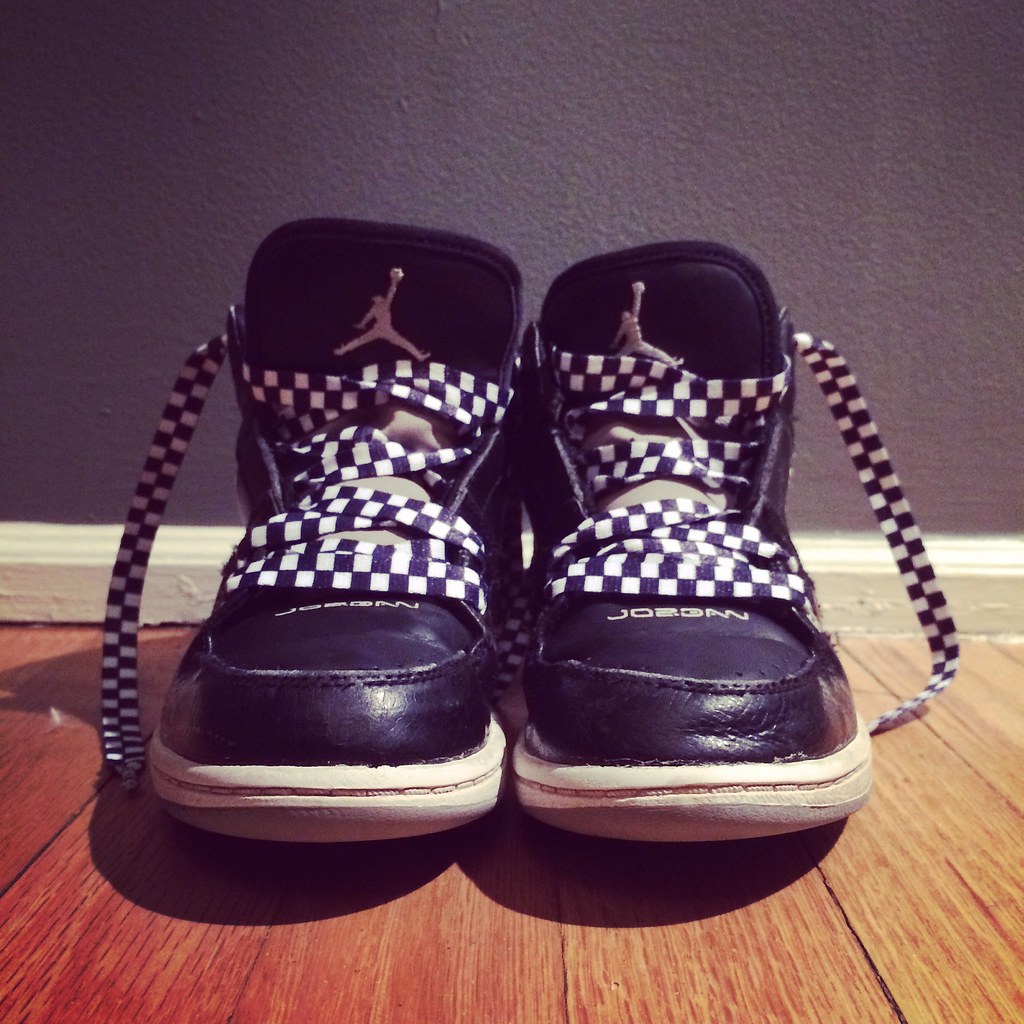The image captures a pair of well-worn, black Leather Air Jordan sneakers positioned at floor level on a brown wooden floor. The shoes are placed against a dark gray wall accented with white trim. The front of the sneakers features the word "Jordan" written in white letters. The shoes have black and white checkered shoelaces, which are loosely laced in a crisscross pattern to facilitate easy wearing. The tongues of the sneakers prominently display the iconic Air Jordan Jumpman logo of a man leaping with legs spread wide and reaching for a ball. The tongues appear to be made of a different material, possibly a grayish-white color, slightly peeking out through the laces. The shoes cast subtle shadows on the wooden floor, adding depth to the scene.